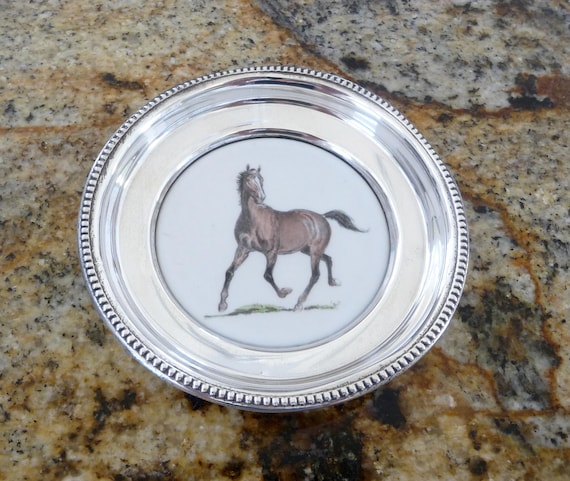This photograph captures a small, decorative silver plate with intricate embellishments along its textured edge, featuring tiny dots. The centerpiece of the plate depicts a dynamic scene of a brown horse, identified as a pony by some, captured in mid-trot. The horse’s mane and tail, depicted in flowing black, suggest movement as if blowing in the wind. It appears to be moving over a patch of grass against a white background. The plate rests on a speckled granite countertop with tones of beige, tan, brown, and black, likely situated in a kitchen. The entire image is framed in a square format, emphasizing the plate’s detailed features and its elegant setting.